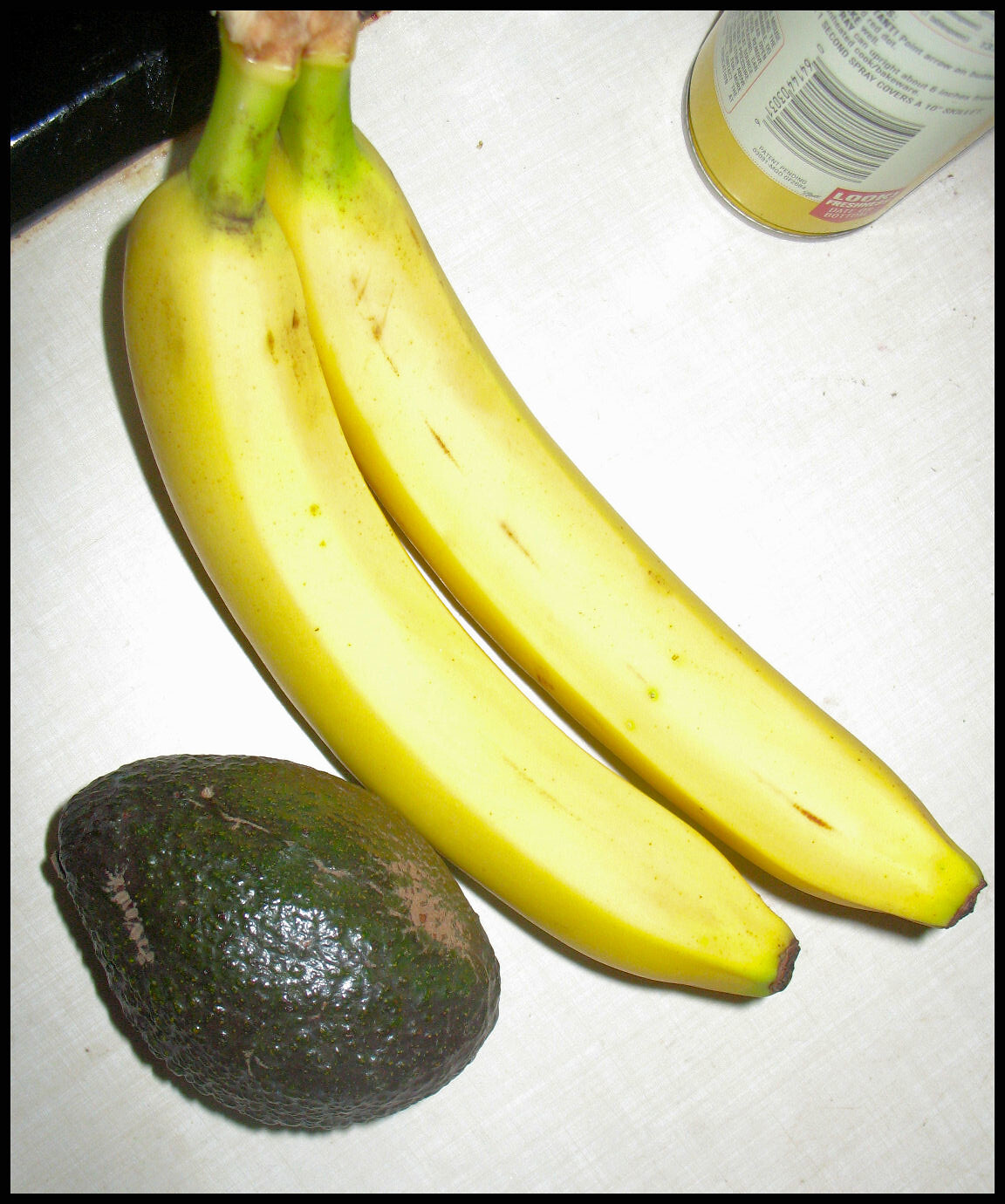In this close-up photograph, a very ripe avocado displaying light brown splotches and dark green-brown bruising is prominently featured on a countertop. The avocado is positioned adjacent to two impeccably ripe bananas, whose slightly green, partially cropped stems hint at their freshness. Directly above the bananas, a section of black metal suggests the presence of a stove top or tile work. To the upper right, around the two o'clock position, there is an aerosol can, possibly SPAM, PAM, or another type of canned good, adding to the assortment of items on the counter. The countertop itself is a light gray or white tile, providing a neutral backdrop that highlights the vibrant colors and textures of the fruits and objects.